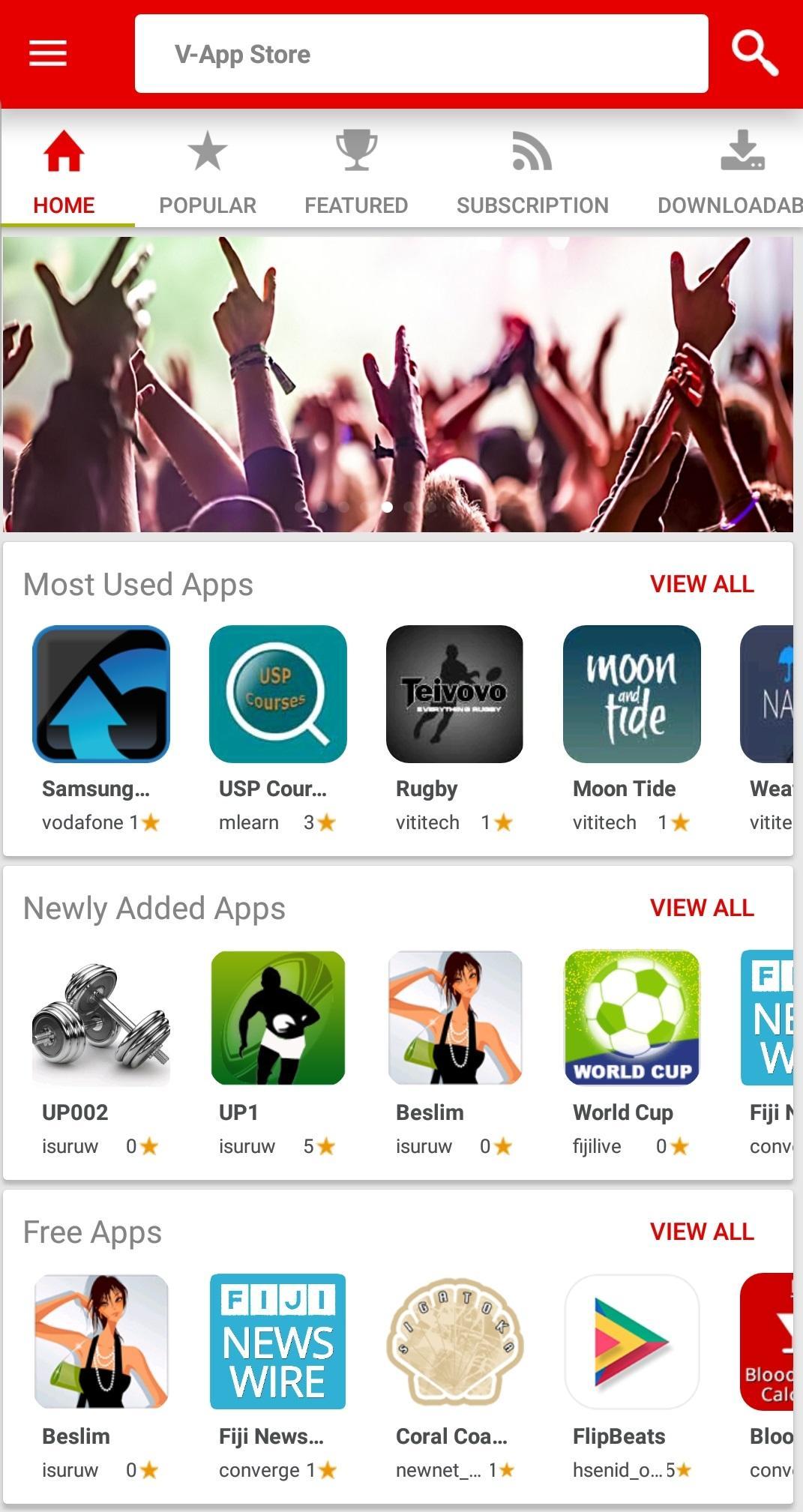The mobile website showcases the App Store, prominently displayed at the top against a red background. A search bar is situated just below, accompanied by a hamburger menu on the far left. Beneath this, a white navigation strip is laid out horizontally, featuring labeled icons for Home, Popular, Featured, Subscription, and Downloaded.

In the middle section, a dynamic concert scene unfolds with hands raised high, capturing the energy of a live performance. Directly beneath this image, a section labeled "Most Used Apps" displays a grid of various app icons, including Samsung, Vodafone, USP, Rugby, and Moon Tide.

Continuing further down, there is a segment for "Newly Added Apps" highlighted by an assortment of app names such as UP002, UP1, Besley, World Cup, and Fiji something (the rest of the text is unclear).

The webpage concludes with a "Free Apps" section, showcasing available apps like Besley, Fiji News, Coral Coast, and Flipbeats, offering users a diverse selection to explore and download.